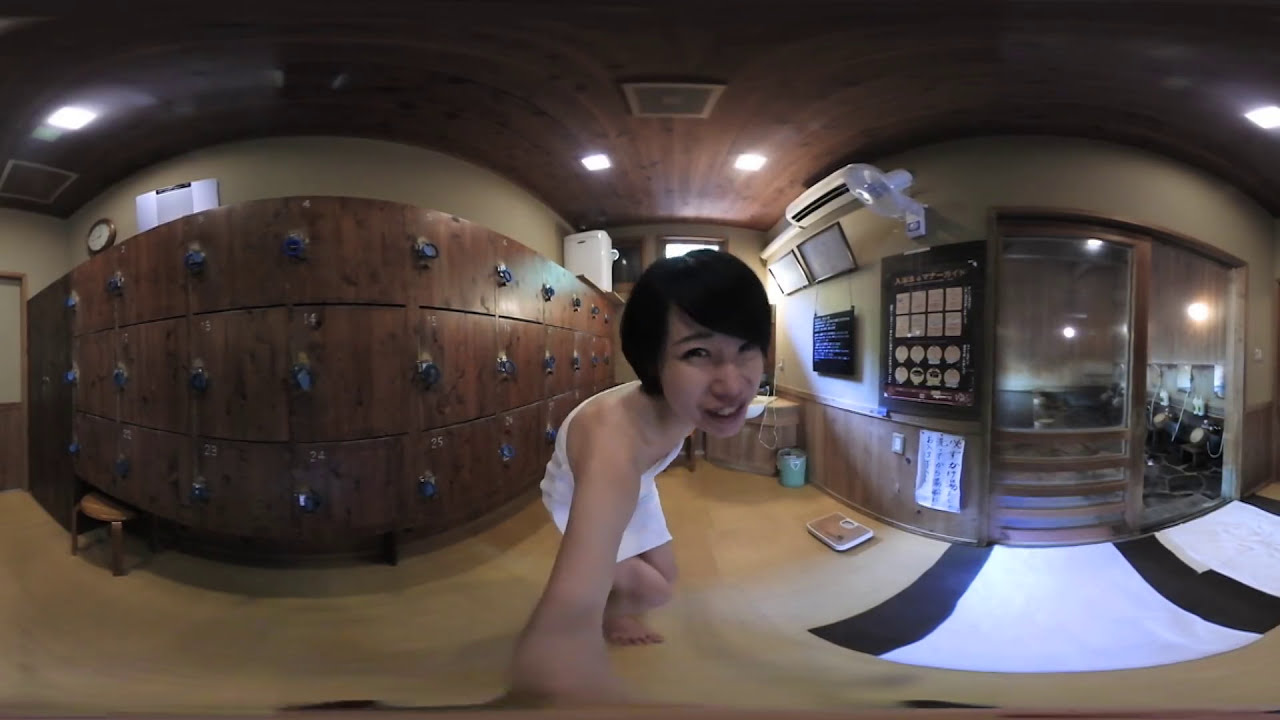In this detailed image, we see a young Asian woman with short brown hair, smiling and seemingly enjoying herself, wrapped in a white towel, inside a spa setting. She's barefoot and hunched slightly as she holds the camera in her right hand. The spa room is characterized by its distinct architectural elements: a curved wall of wooden lockers with locks on the left side, a polished dark wood ceiling adorned with pot lights and a vent, and a couple of white and black-lined mats on the right side. The tan floor features a scale, suggesting a focus on health and wellness. Also noticeable are a variety of sauna-related items, including a heater, a hanging heater, and two TV monitors situated to the left. The image also shows a glass double door or sliding door with signage and posters on the right, likely in Japanese. The overall ambiance, accentuated by the panoramic shot, exudes a warm and inviting atmosphere typical of a well-appointed spa.